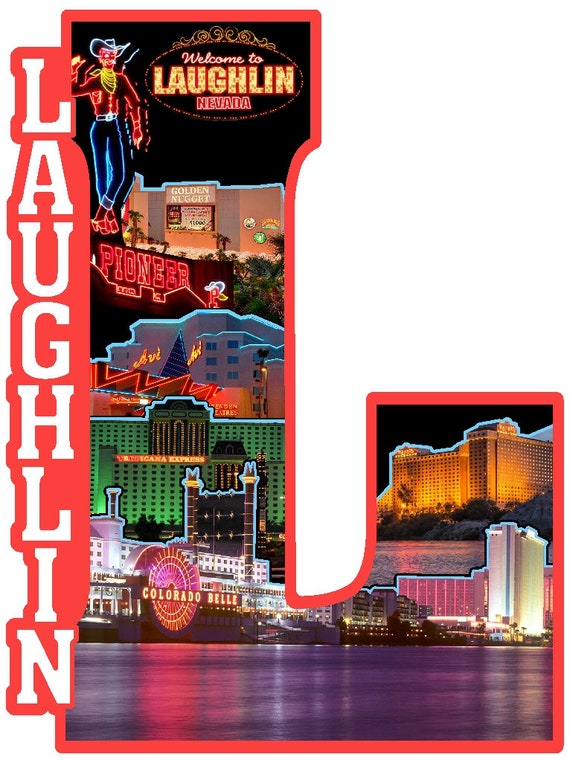The image is of a large, red-outlined "L" sticker, reminiscent of a souvenir shop item. This "L" is filled with a collage of lively, neon-lit photographs showcasing the cityscape of Laughlin, Nevada. At the top of the "L," there's a brightly colored welcome sign stating "Welcome to Laughlin, Nevada," accompanied by a cartoonish, neon-lit cowboy figure. Below this, you'll find an advertisement for the Golden Nugget, followed by a red neon sign for the Pioneer, possibly a prominent restaurant or establishment in Laughlin.

Descending the "L," the collage features various illuminated buildings, including a brightly lit hotel with green neon lights labeled something express, and a riverfront scene with the Colorado Belle paddle boat, which could be either a restaurant or situated on the waterway itself. As the "L" curves, there is a large hotel with gold lighting, surrounded by water and additional high-rises including a pink-colored motel.

Running vertically along the exterior left side of the "L," the word "Laughlin" is spelled out in white block letters with the same red outlining. The entire design serves as an elaborate advertisement for Laughlin, Nevada, emphasizing its vibrant nightlife and array of attractions.